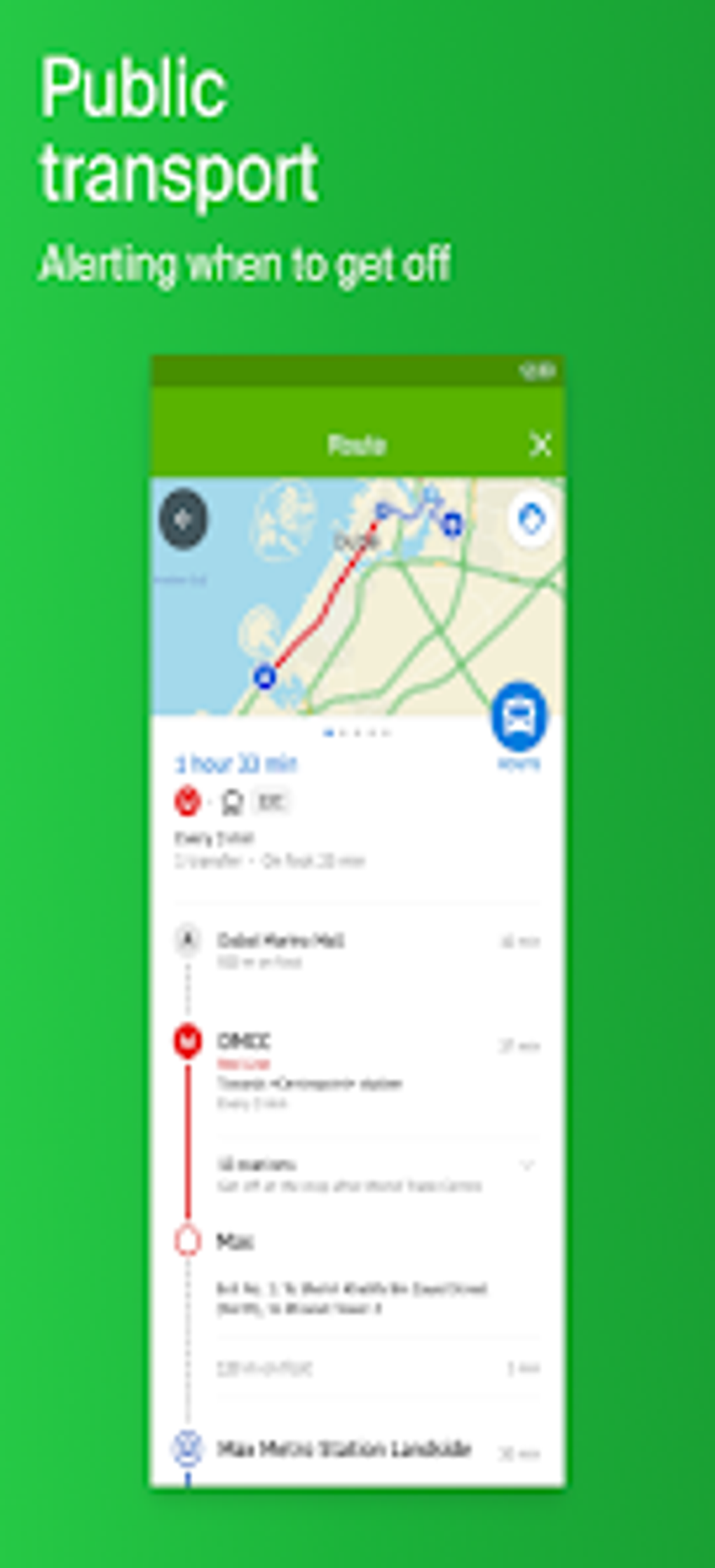The image is a low-resolution screenshot of an advertisement designed for mobile devices, featuring vertical orientation. The overall background is a standard shade of green. In the top left-hand corner, there is white text that reads “Public Transport,” with the subtext “Alerting When to Get Off” below it. 

Embedded within the larger image is a screenshot of a mobile device display, also oriented vertically. The upper portion of the display includes a dark green bar, followed by a lighter green bar containing some white text. Below these bars is a map feature, where the top left section shows a blue body of water, likely an ocean or lake, while the right section depicts a gray landmass intersected by green roads.

A highlighted path connects two blue points along the coast, indicating a route with a duration of three hours and thirty-three minutes, suggesting this could be a train ride. Additional instructions are provided below the map, offering details on how to reach the destination and the estimated travel time.